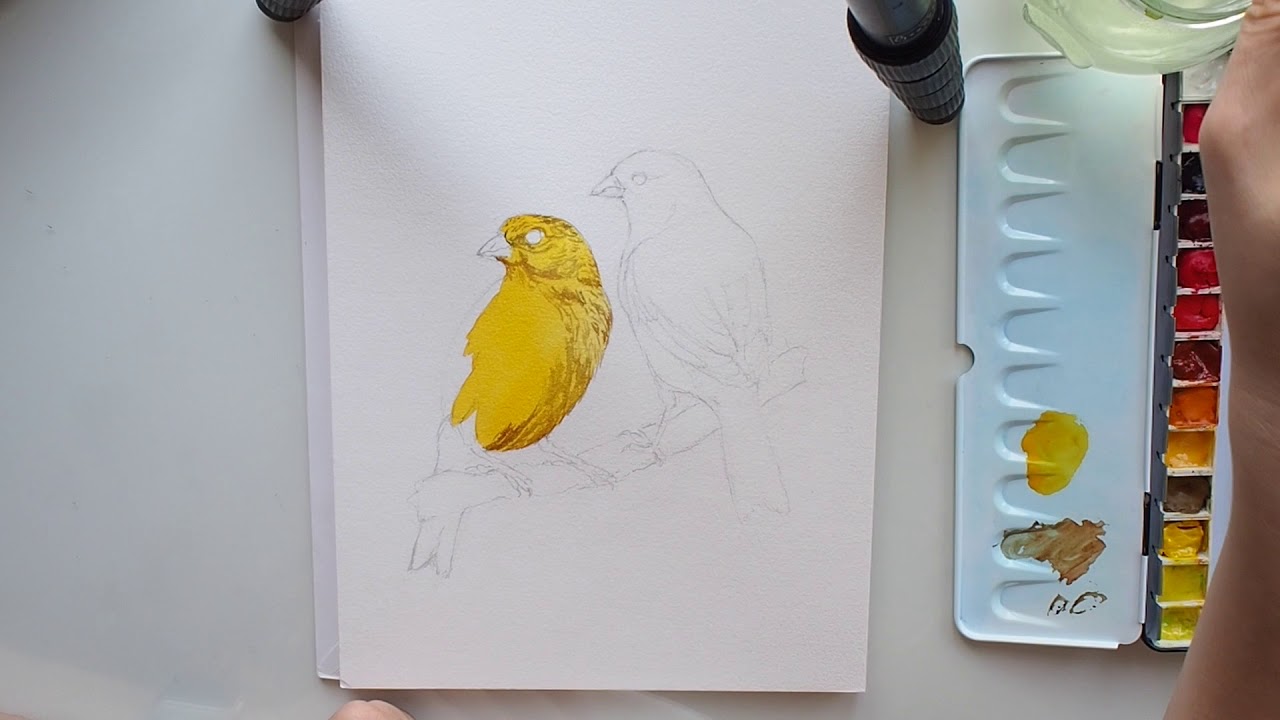In this detailed image, we see an artist in the process of creating a watercolor painting, centered on a plain white piece of paper resting on a white countertop. The paper features a detailed pencil sketch of two birds standing on a branch. The bird on the left has begun to be filled in with a mustard-yellow paint, accented with brown, though its beak, feet, and eye remain uncolored. The bird on the right and the branch are only in pencil outline, showing no signs of paint yet. To the right of the image, the artist's hand is visible, reaching into a watercolor palette. This palette contains various shades predominantly in reds, browns, oranges, and yellows, with a specific section for testing colors. Additionally, a bottle of paint or possibly water is positioned in the upper right corner of the scene. The overall composition emphasizes the process and tools of the artist as they bring the piece to life.